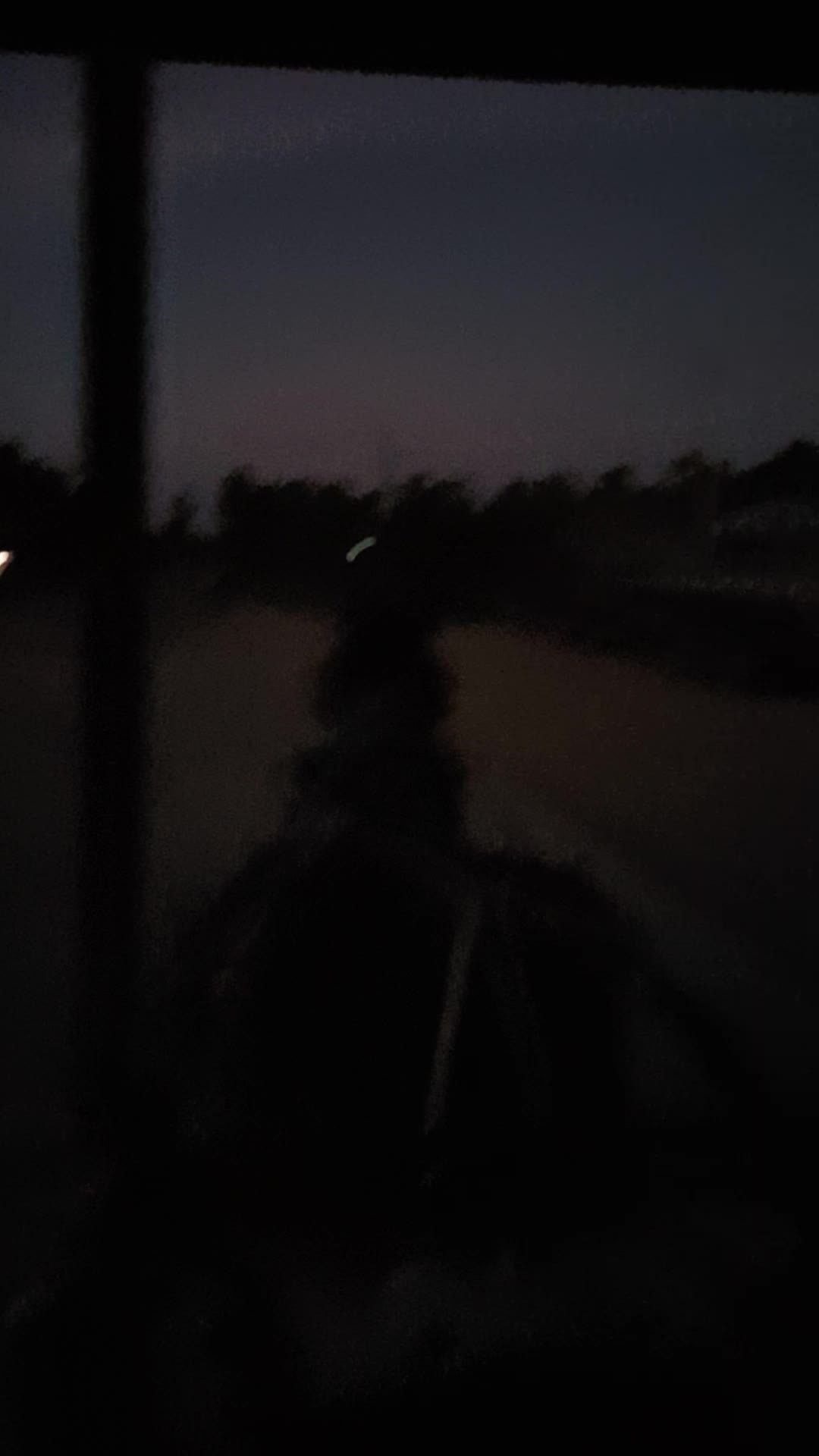The photograph is a dark, dimly lit image that appears blurry, taken either at dusk or dawn. The composition is vertically elongated, about two and a half to three times as tall as it is wide. You're looking at a scene framed by a possible doorway or window. To the left of the image, a vertical bar, resembling part of a window or door frame, runs up and down with a 90-degree angle at the top, suggesting a corner or sill. The sky transitions from a subtle pink hue just above the tree line to shades of light and then medium blue, indicating the remains of daylight fading or the early light of dawn.

In the background, a silhouette of a tree line extends across the image, providing the only clear shapes against the sky. Central to the scene is a slightly ambiguous, snowman-like shape below the tree line, which might be a statue or even a fountain with the suggestion of water illuminated by a faint light. On either side of this shape and below the tree line, there could be water bodies such as a lake or river, adding to the dreamy, reflective atmosphere. Together, the elements evoke a somber, tranquil imagery viewed from inside looking out, possibly from a boat or a quiet lakeside window.